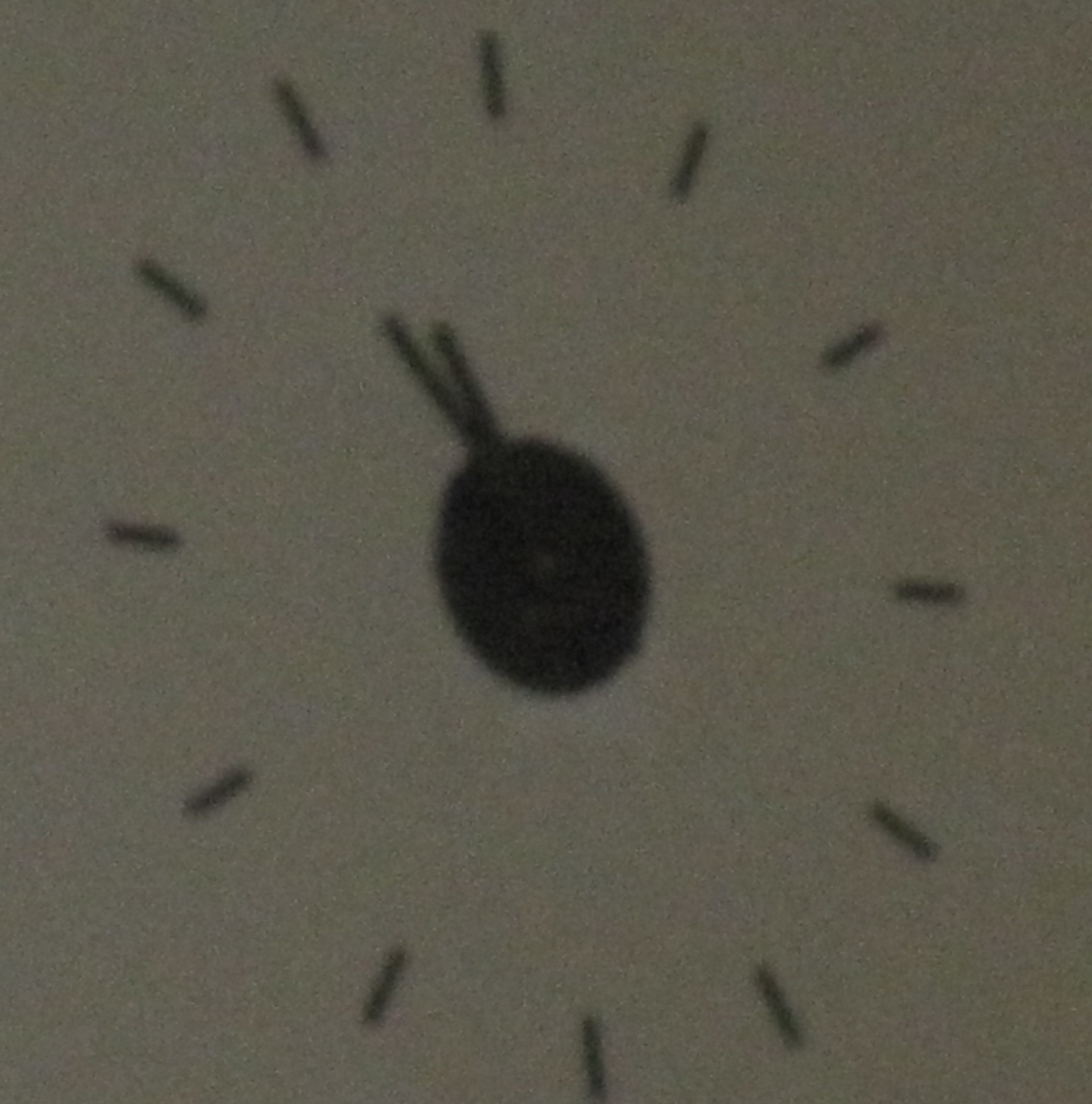This photograph depicts a close-up of a somewhat blurry and grainy clock face with a white background that appears as a dark gray due to the image's overall low quality. The clock has a solid black circle at its center. Two very short, dark black hands are positioned such that the hour hand is pointing at the 11 and the minute hand is slightly before the 11, suggesting the time is approximately 10:55. The clock features simple hash marks in place of numbers. The heavy graininess of the image results in noticeable pixelation, with tiny black and white dots scattered across the surface, and the close-up nature of the photograph obscures the clock's housing and any external numbers.